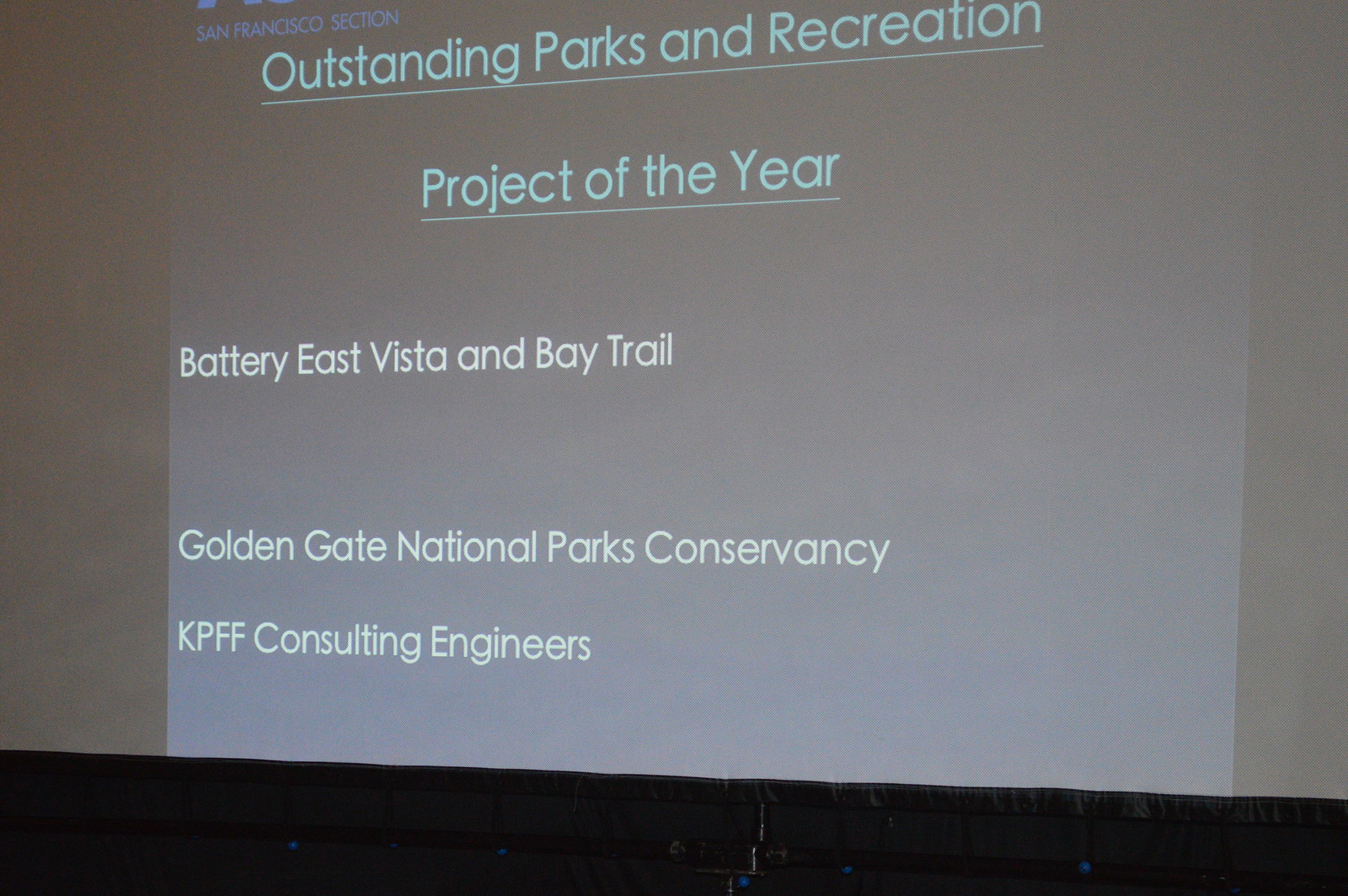This image captures a detailed close-up of a projector screen dominated by a dark blue presentation slide against what appears to be a white wall. The screen's content includes various shades of blue and white text. At the very top, in light blue text, it reads "Outstanding Parks and Recreation Project of the Year." Beneath this, aligned to the left, in white text, are the project details: "Battery East Vista and Bay Trail, Golden Gate National Parks Conservancy, KPFF Consulting Engineers." Notably, there is additional space between "Battery East Vista and Bay Trail" and "Golden Gate National Parks Conservancy." The bottom part of the image shows a black section, likely indicating either the wall or empty space below the screen. The overall presentation appears formal and straightforward, emphasizing the recognition of the Parks and Recreation Project of the Year.